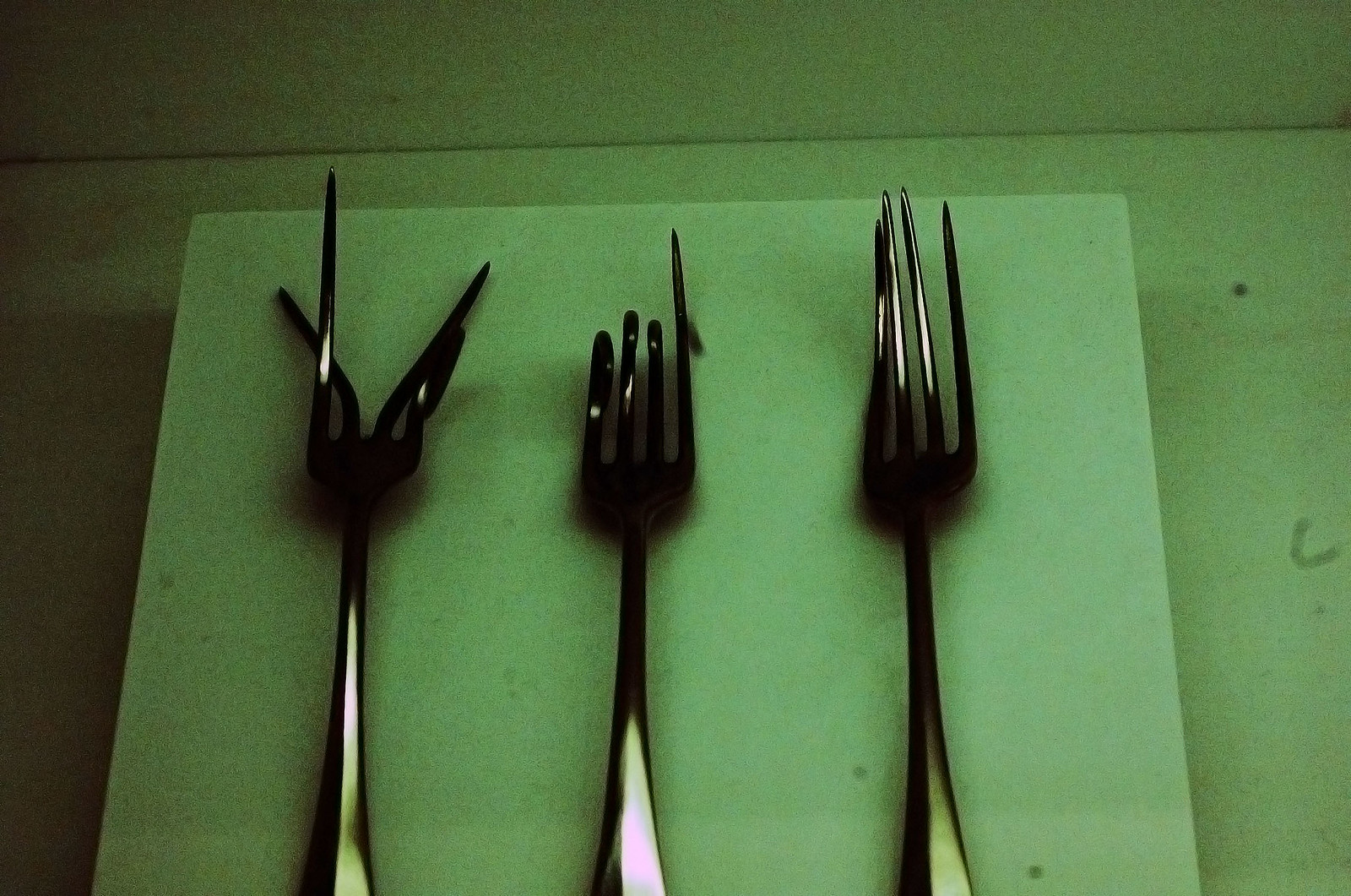In this dark, underexposed photograph, three metal forks are aligned in a row on a slightly elevated, whitish-green background. The low-quality image, marred by heavy grain and washed-out colors, features forks noticeably damaged and deformed. Each fork is orientated with its handle facing downwards and prongs directed upwards.

The leftmost fork stands out with its four tines splayed dramatically—two curving to the left, one pointing upwards, and the second from the left bent beneath at a 45-degree angle to the left. The middle fork has an unusual configuration with one notably straight tine on the right and the remaining three distorted in various directions. The rightmost fork also has four tines, all of which are bent and damaged, with one prong curling slightly upwards.

Set against a green background that complements their muted, dark appearance, the forks seem to be on a napkin or paper over a larger green surface, creating the impression of an artistic and intentional display of wear and tear. A closer inspection reveals that the background is slightly dirty and textured, emphasizing the forks' dilapidated condition. The intriguing composition and unusual presentation hint at an artistic or experimental intent, despite the image's dark and grainy execution.